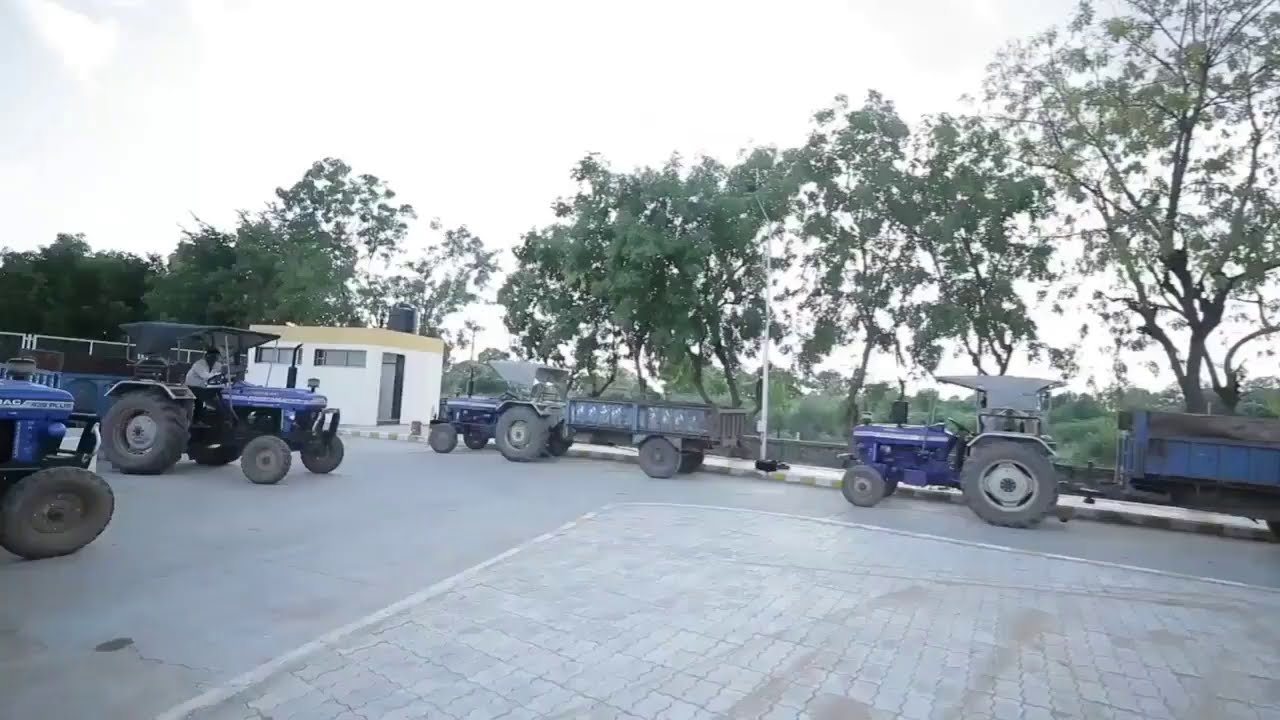The photograph captures a somewhat cluttered parking area or clearing, featuring several types of farming vehicles and equipment. The ground in the foreground consists of gray cobblestones, while further back it transitions to a smoother, gray asphalt surface. There are at least four navy blue or indigo tractors scattered throughout the scene, two directly in front of the camera, two more towards the left, and one partially visible peeking from the left edge of the image. These vehicles appear well-used, indicated by the dusty wheels. Some of these tractors have attached trailer beds, with one notably longer hauler. A driver can be seen sitting in one of the smaller buggies. The setting suggests either an industrial site or a military operation, although this isn't entirely clear. The background is bordered by sparsely but large green-leaved trees, adding a natural backdrop to the otherwise mechanical scene. Adjacent to these trees, a small white shed or guard shack is visible, further contextualizing the area. The sky overhead is a dull, light gray, hinting at overcast conditions without direct sunlight. The photograph itself is slightly skewed, with the sunlight entering from the left, creating an uneven composition.